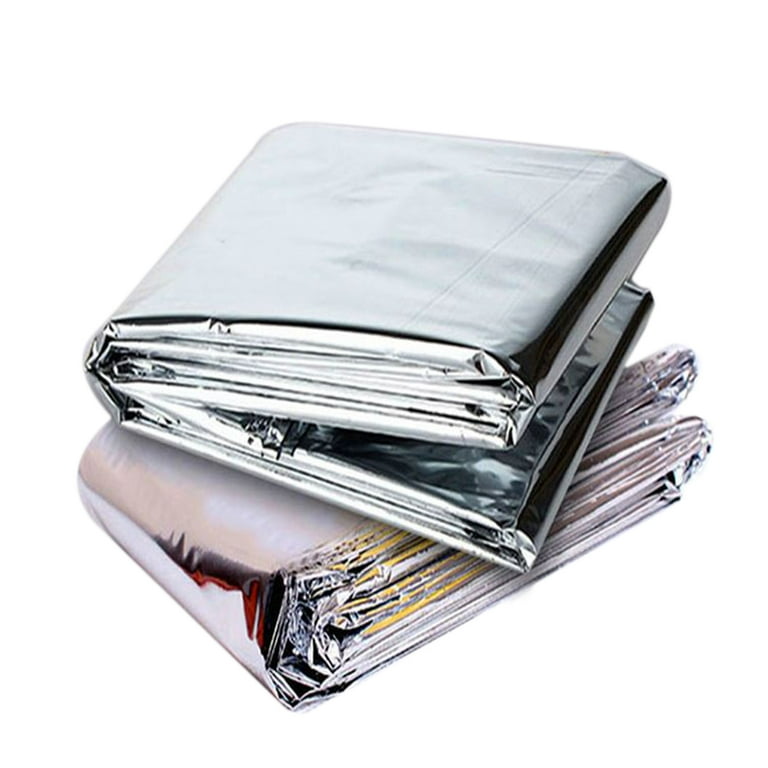This advertisement features a photograph of two meticulously folded, shiny silver materials, likely space blankets or mylar sheets, placed against a seamless white background. The two items are folded so neatly and precisely that they resemble closed wallets or cube shapes, with intricate, dark creases and wrinkles throughout. The top sheet exhibits a cool-toned silver, while the sheet beneath it shows warmer tones, reflecting hues of red, cream, pink on the left side, and yellow on the right. Both sheets are offset, with the open fold of the top sheet facing the bottom right of the image, and the bottom sheet's fold directed towards the top right. The precise presentation and layered arrangement highlight the detailed craftsmanship of these potential emergency blankets, making them appear impeccably organized and distinctly separate despite their close stacking.